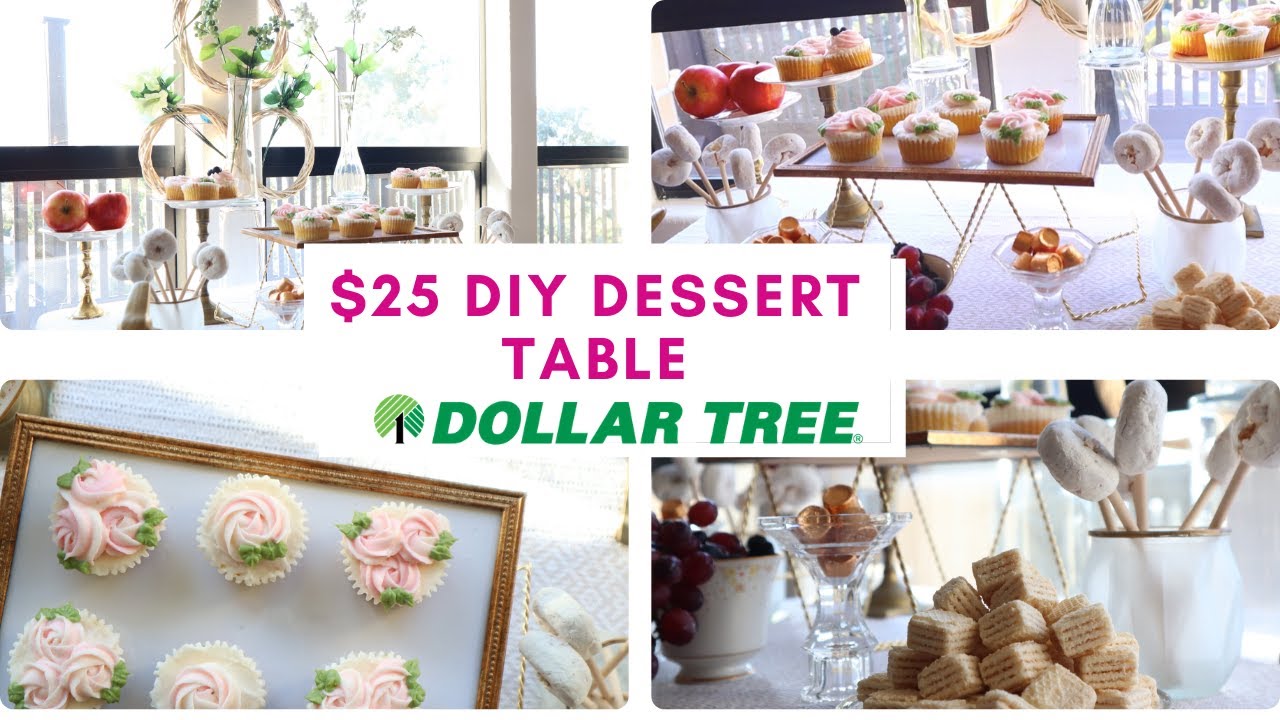The advertisement is a collage of four vivid images centered around a budget-friendly, $25 DIY dessert table, showcasing how to create appealing dessert arrangements using items from Dollar Tree. The central text reads "$25 DIY Dessert Table" in bold reddish font, with the Dollar Tree logo and text in green beneath it.

Each of the four images highlights different elements of the dessert table setup. One image features delectable cupcakes adorned with pink swirls of frosting and a touch of green garnish. Nearby, a glass jar and a larger round vase filled with fruit—likely grapes—add to the display's elegance. Another image captures a variety of cookies positioned at the bottom right, alongside a mixture of cupcakes, apples, donuts, and green plants in vases, creating a lush array of treats. Yet another image zooms in on an assortment of cupcakes, apples, and other desserts, further emphasizing the diverse and colorful options available for crafting an inviting dessert table—presumably all available at Dollar Tree.

This detailed and visually appealing arrangement demonstrates how to create a stylish and varied dessert table on a budget, using easily accessible items.